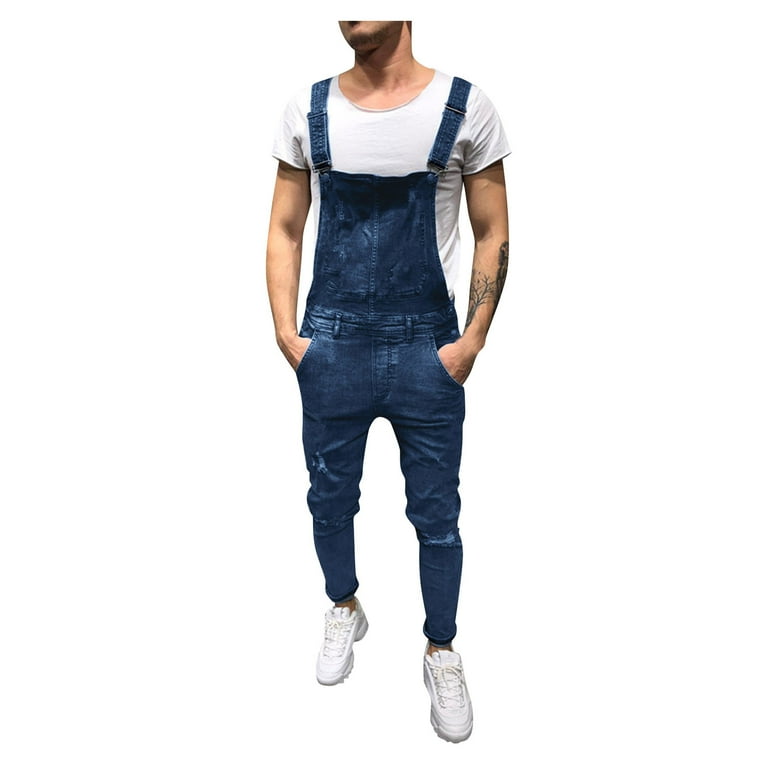This image features a young Caucasian man, likely aged between 18 and 30, posing in front of a completely white background. His face is partially obscured, cutting off from just above his lips, but revealing a chin with a bit of stubble. He has brown hair, or it might be a shadow. The focus is primarily on his attire, which consists of a pair of well-fitted, full-length denim overalls rolled up slightly at the ankles, worn over a white scoop neck t-shirt. Both straps of the overalls are securely fastened over his shoulders, and the fabric appears relatively new and unworn. His hands rest casually in the overalls' waist pockets, revealing tattoos on his left forearm, one depicting a tree and another indiscernible design near the elbow. Completing his outfit are bright white tennis shoes, possibly worn without socks or with short athletic ones. The overall scene suggests a photo shoot or magazine spread, with all background elements removed to emphasize his clothing.